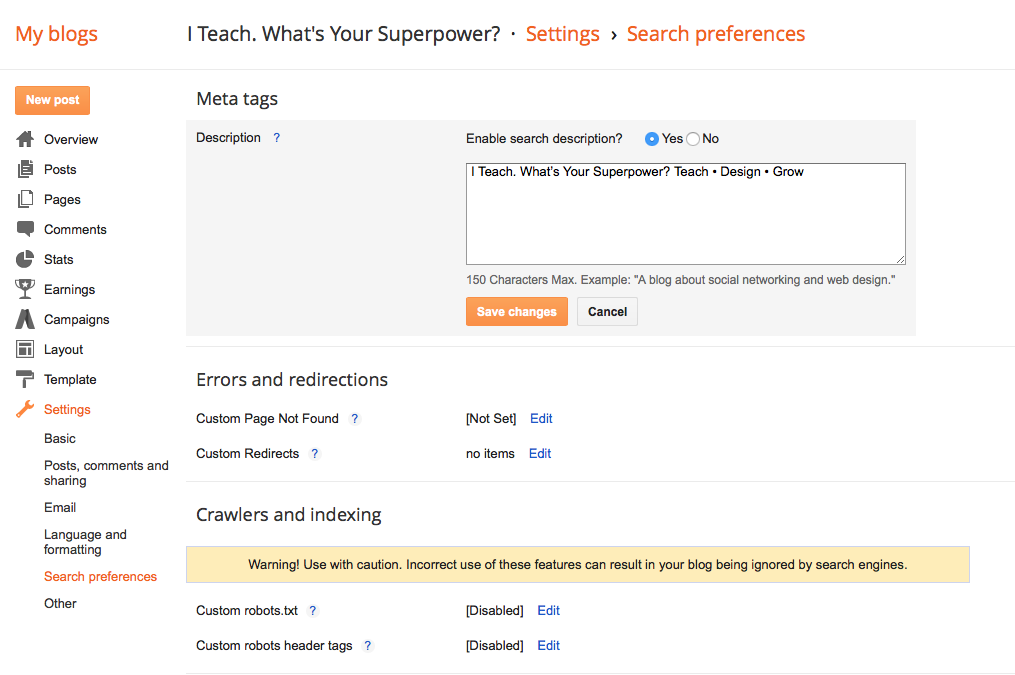Screenshot of a Blogger Dashboard - Detailed Description:

The image appears to be a screenshot from a Blogger dashboard webpage. 

In the upper left-hand corner, there is a section titled "My Blogs" written in red text. Directly below this title, there's an orange button labeled "New Post."

A vertical list of menu items is displayed in black, each accompanied by a corresponding black icon. The menu items include: Overview, Posts, Pages, Comments, Stats, Earnings, Campaigns, Layout, Template, and Settings. The "Settings" option is highlighted in orange, indicating it is currently selected. 

Under the "Settings" menu, a sub-list is visible with the following items: Basic, Posts, Comments and Sharing, Email, Language and Formatting, Search Preferences (highlighted in orange), and Other.

To the right, at the top of the screen, there's a heading in black text that reads, "I Teach, What's Your Superpower?" Below this, the text "Settings - Search Preferences" is displayed in orange.

The main content area beneath this heading features various options related to preferences for the blog:
- A section titled "Meta Tags" includes a descriptor with the option "Enable search description" set to "Yes." Within a text box, the phrase "I Teach, What's Your Superpower? Teach, Design, Grow." is entered. A note below the text box indicates a character limit of 180 characters, providing an example: "A blog about social networking and web design."
- Two buttons follow this section: an orange "Save Changes" button and a "Cancel" button.

Further down, there is a section for "Errors and Redirections":
- "Custom Page Not Found" is listed as "Not Set" with an "Edit" option available.
- "Custom Redirects" shows "No items" with an "Edit" option available as well.

The next section addresses "Crawling and Indexing." Here, there is a yellow rectangle with a yellow background and black text that reads, "Warning: Use with caution, incorrect use of these features can result in your blog being ignored by search engines."

Lastly, there are options for "Custom robots.txt" and "Custom robots header tags," both of which are currently disabled but have "Edit" options.

This highly detailed visualization organizes all pertinent settings and warnings, providing a comprehensive overview of the blog's configuration tools.